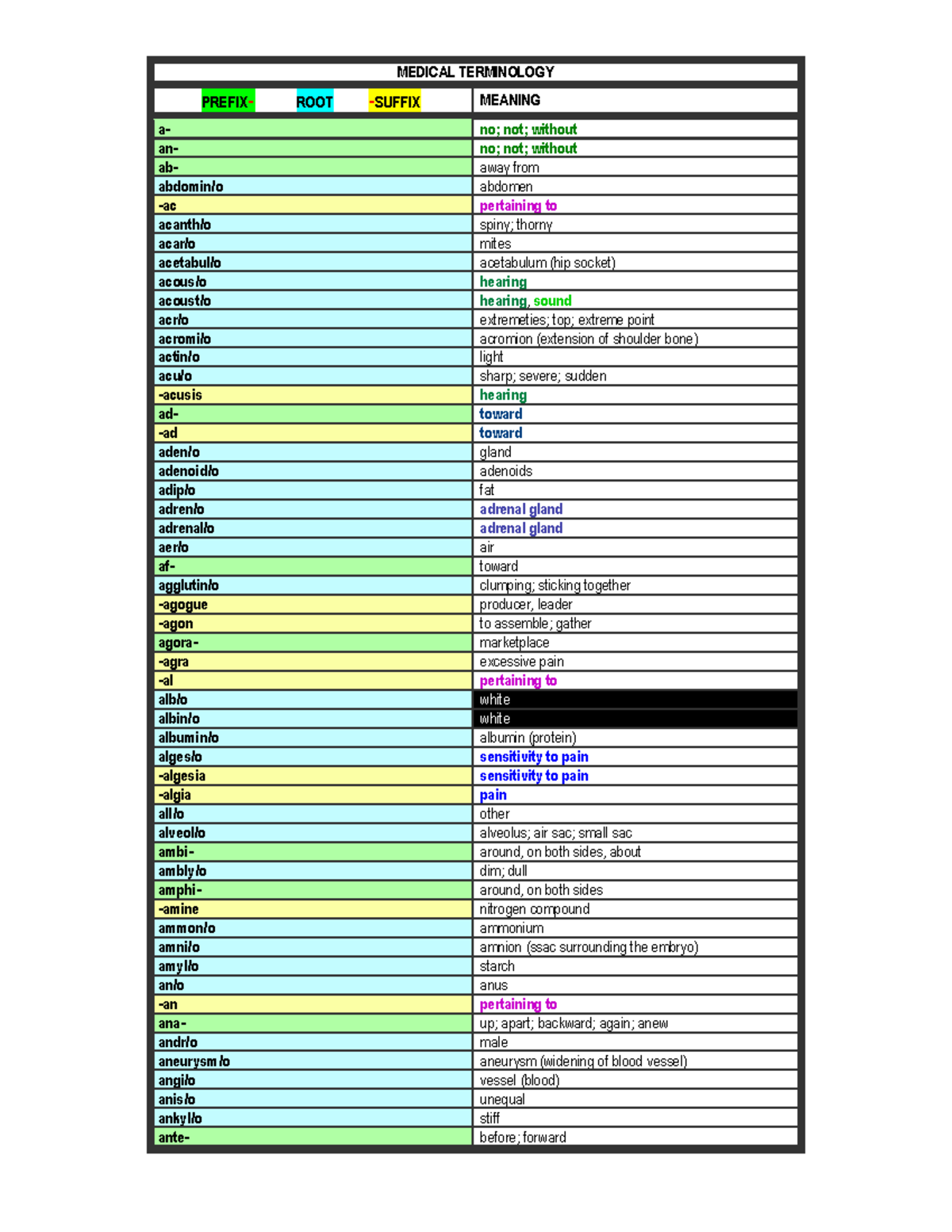This image features a meticulously organized page dedicated to medical terminology, prominently labeled "MEDICAL TERMINOLOGY" at the top in bold, uppercase letters. The page is framed by a clean black border and structured into two distinct columns, each serving a different purpose.

On the left side, a single column lists various medical prefixes, roots, and suffixes. These categories are identified by color-coded headers: "Prefix" in green, "Root" in blue, and "Suffix" in yellow. The terms displayed include "a", "an", "acantho", "acro", "ario", "albino", and "ante", among others. Each term is highlighted in its respective section color: for example, "a" in green for Prefix, "ac" in blue for Root, and "ad" in yellow for Suffix. This color-coding is consistently applied throughout the list, aiding in quick identification and categorization.

The right side of the page features another column labeled "Meaning" in black type. This section provides clear, concise definitions for each of the terms listed in the left column. For instance, the term "a" in green is defined as "no, not, without." The term "acuso," highlighted in blue, is defined as "hearing," while "acusis," in yellow, also means "hearing." Additional definitions include "algiso" (sensitivity to pain), "allo" (other), "ambi" (around, on both sides, about), "anno" (anus), and "anna" (up, apart, backward, again, new).

Each term from the left column is systematically paired with its corresponding meaning in the right column, creating a comprehensive and visually intuitive guide to understanding medical terminology.